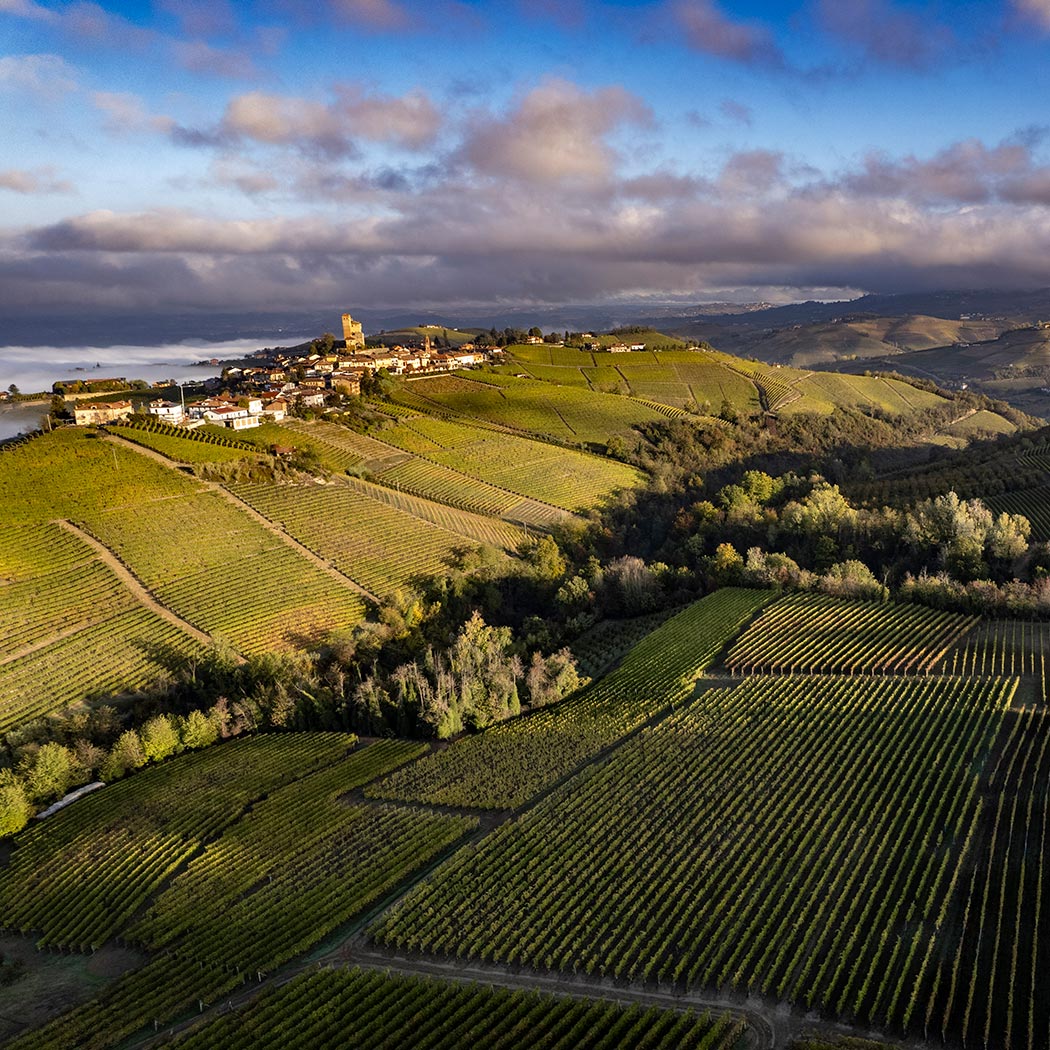This stunning aerial photograph captures the vast and meticulously organized countryside farmland. The landscape features lush, green fields, neatly divided into sections with long, precise rows of crops, possibly vineyards or other green plants. Between two prominent hills, a line of natural green trees provides a beautiful contrast to the cultivated land. The hills are dotted with approximately twenty small houses, each with a brown roof, nestled on the far hilltop. The horizon showcases a picturesque mountain range, bordered by a blue sky with scattered clouds casting shadows on the terrain below. Toward the edge of the image, a serene harbor with blue water suggests the presence of the ocean, and a small village with white to reddish-tan buildings lies along the coast, adding to the scenic beauty of this breathtaking countryside view.